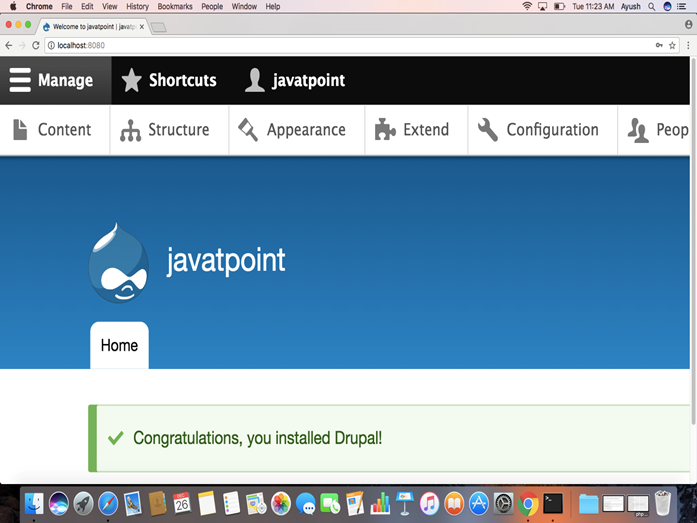A detailed screenshot of a webpage displayed in Google Chrome on a Mac computer. At the very top, the menu bar includes the labels Chrome, File, Edit, View, History, Bookmarks, People, Window, and Help, alongside the Apple logo. Below this menu bar is the browser's address bar, featuring the input URL "localhost:8080", and to its right are buttons labeled Manage, Shortcuts, and JavaPoint.

The main portion of the screen is occupied by a web application welcome page for "JavaPoint." A horizontal navigation menu below the search bar lists sections labeled Content, Structure, Appearance, Extend, Configuration, and People (with the word "People" slightly cut off). 

The central area of the screen has a rectangular blue background with the text "JavaPoint" displayed in white at the top. Beneath this is an icon depicting a simple cartoon face with two eyes, a nose, and a mouth, above the word "Home." A prominent light green bar stretches across the screen with the message "Congratulations, you installed Drupal." Below this are various colorful notification icons typically seen on a computer's desktop environment, indicating a range of available functions and alerts.